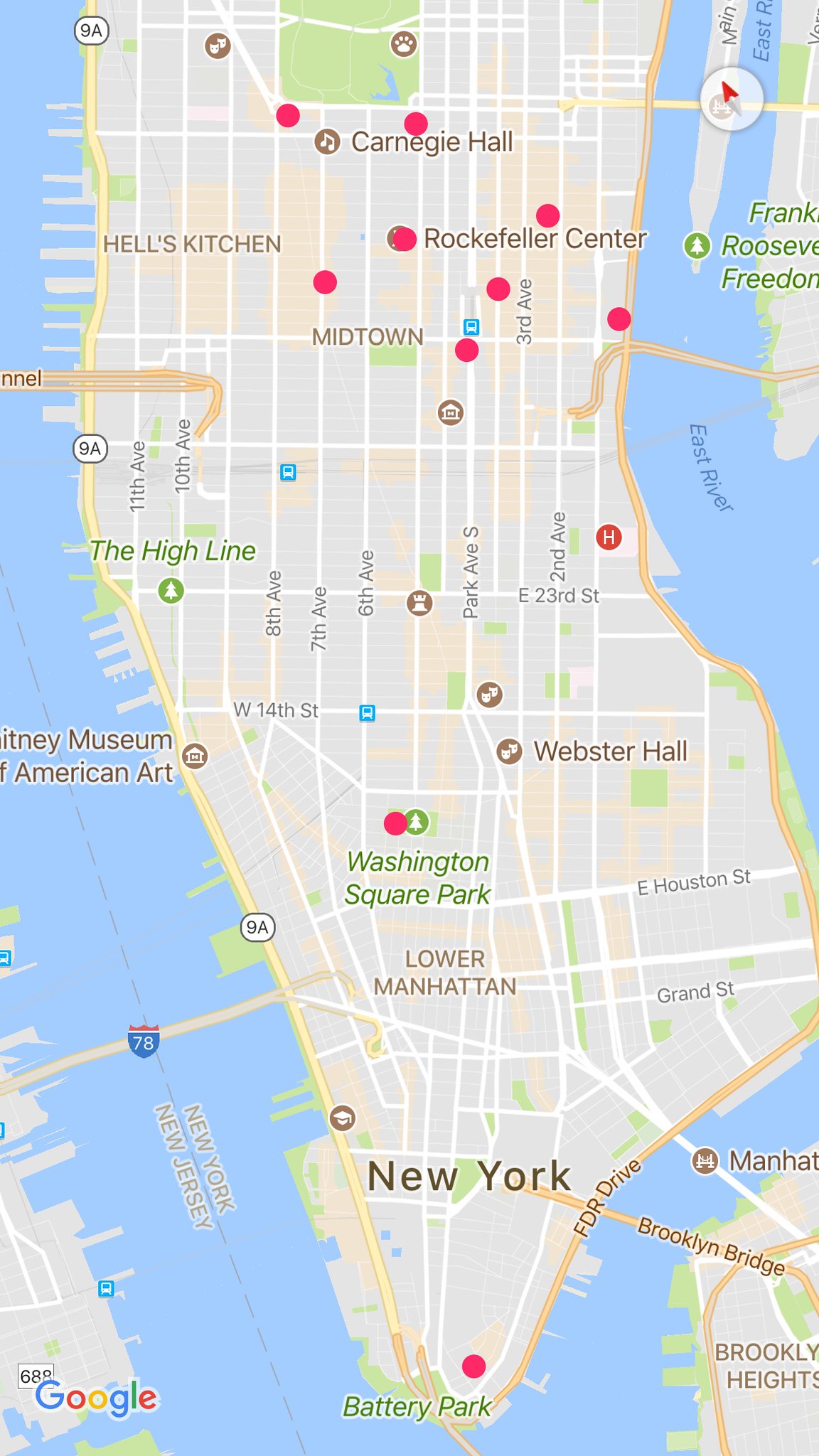This image showcases a digital map, likely viewed on a phone or computer, designed to help users navigate or locate specific destinations in New York City. The background is predominantly blue, while a large gray mass represents the city. Scattered across this map are numerous red dots indicating notable landmarks and destinations.

At the top section of the map, near some of these red dots, Carnegie Hall is prominently labeled. To the left, in brown text, the area known as Hell's Kitchen is identified. Moving to the right, Rockefeller Center is marked alongside a long white line denoting Midtown. 

The map also highlights major avenues such as 8th Avenue, 7th Avenue, and Park Avenue South. One particular location, Washington Square Park, is denoted with a red dot and a green circle, accompanied by green text just beneath.

In the lower part of the map, brown text labels the area as Lower Manhattan, while black text near the bottom simply states New York. Further down is another red dot next to the text for Battery Park. To the left, against the blue background, is another New York, New York label, along with an interstate sign with the number 78 positioned below it.

In the lower left corner of the image, the Google logo is visible with its distinctive blue "G", red "O", yellow "O", lowercase blue "g", green "l", and red "e" typography.